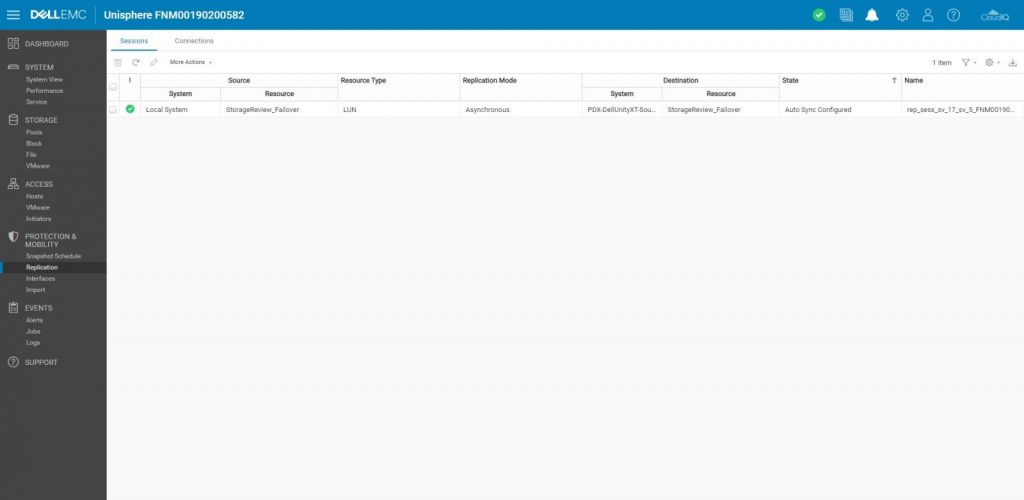**Caption: Detailed View of Dell EMC Unisphere Interface**

The image displays a detailed screenshot of the Dell EMC Unisphere web interface. At the top, a blue navigation bar prominently shows the label "Dell EMC" along with a menu icon. The label "Unisphere" is also visible, along with a unique identifier "FNM 00190200582." On the right side of this top bar, there is a green circle with a check mark, indicating system health or status, accompanied by icons for notifications, settings, profile, and help.

Running down the left-hand side of the interface is a vertical column containing several menu options: "System," "Storage," "Access," "Protection and Mobility," "Events," and "Support." Each of these main menu items has sub-items listed beneath them, although the text is too small to be legible.

To the right of this column, the interface displays sections for "Session" and "Corrections," with associated icons for refreshing, editing, and additional actions. Below this, the layout comprises various headers including "Source," "Systems and Resources," "Local System," "Resource Type" (LLN), "Replication Mode" (Asynchronous), "Destination," "System," "Resource" (CDX), "Storage State," and "Name" (Autosync), capturing detailed configurations and states of resources.

This thorough depiction highlights the complex and comprehensive nature of the Dell EMC Unisphere management interface, displaying various system statuses and management options in a structured format.